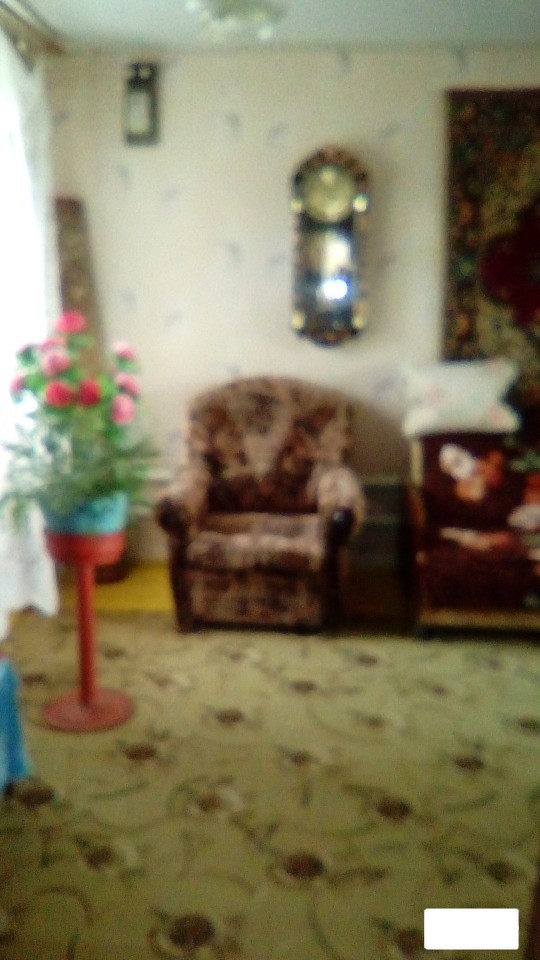In this photograph, albeit blurry, an old-fashioned living room is depicted with great nostalgia. The room features off-white walls adorned with sparse blue or purple feather-like patterns. Dominating the center of one wall is a substantial wall clock, occupying roughly a third of the wall's length. To the left of the clock, near the ceiling, sits an unidentified black rectangular object, while a painting hangs to the clock's right. Beneath the clock, a brown armchair with a subtle pattern on its fabric is positioned. Adjacent to the chair is a modest chest. The floor is partially covered by a beige rug, embellished with brown floral designs. On the left side of the room, sunlight filters through sheer drapes that hang over a window. A red flower stand, bearing a turquoise blue pot filled with flowers (the authenticity of which is uncertain), stands proudly in front of the window. The room's ambiance is gently illuminated by a glass light fixture mounted on the ceiling.